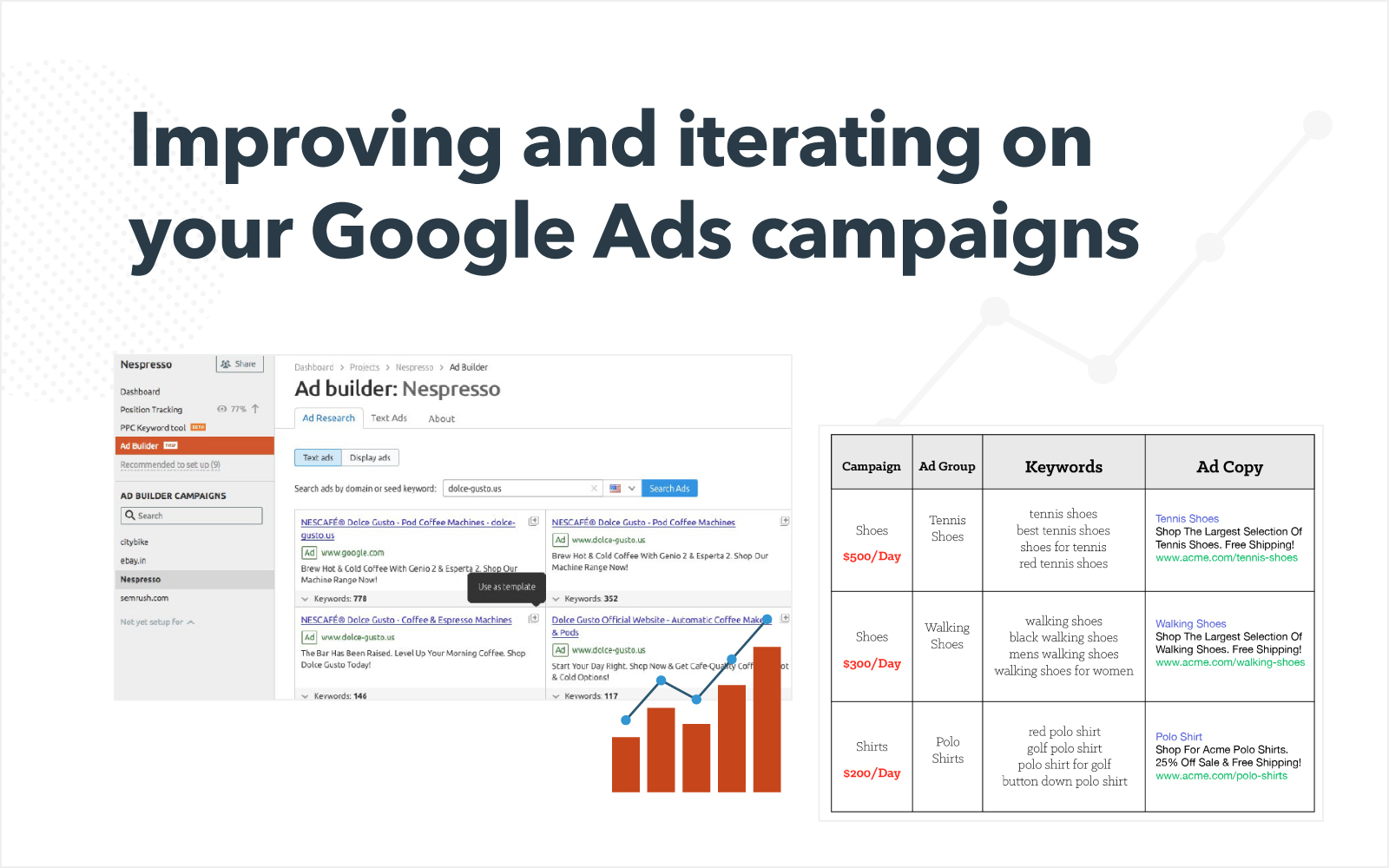The image has a white background with black text at the top that reads, "Improving and Iterating on Your Google Ads Campaign." In the bottom right corner, there is a detailed table with four columns labeled “Campaign,” “Ad Group,” “Keywords,” and “Ad Copy.”

- **First Row:**
  - **Campaign:** 500 per day (written in orange).
  - **Ad Group:** Tennis Shoes.
  - **Keywords:** Tennis shoes, best tennis shoes, shoes for tennis (written in black).
  - **Ad Copy:**
    - **Title:** "Tennis Shoes" (written in blue).
    - **Description:** "Shop a diverse selection of tennis shoes, free shipping."
    - **URL:** www.acme.com/tennisshoes (written in green).

- **Second Row:**
  - **Campaign:** 200 per day.
  - **Ad Group:** Walking Shoes.
  - **Keywords:** Walking shoes, black walking shoes, men’s walking shoes, walking shoes for women.
  - **Ad Copy:**
    - **Title:** "Walking Shoes."
    - **Description:** "Shop a diverse selection of walking shoes, free shipping."
    - **URL:** www.acme.com/walkingshoes.

- **Third Row:**
  - **Campaign:** 200 per day.
  - **Ad Group:** Polo Shirts.
  - **Keywords:** Red polo shirts, golf polo shirts, polo shirts for golf, button-down polo shirts.
  - **Ad Copy:**
    - **Title:** "Polo Shirts."
    - **Description:** "Shop for Acme polo shirts, 25% off sale and free shipping."
    - **URL:** www.acme.com/poloshirts.

On the top left corner of the image, the text "Nespresso" is visible, along with a site menu including options such as Dashboard, Position Tracking, PPC, Keyword Tool, Ad Builder, Ad Builder Campaigns, City Bike, ebay.in, Nespresso, and themebrush.com, with "Nespresso" selected.

On the right side of the image, there is another section with menus labeled "Ad Builder," "Nespresso," "Ad Research," "Text Ad," and "About." Below this, a Google search displays results for "Nescafe Dolce Gusto pod coffee machines." The URLs are google.com, dolce.gusto.us, and three instances of dolce-gusto.us.

At the bottom of the image, there is a paragraph written in orange text.